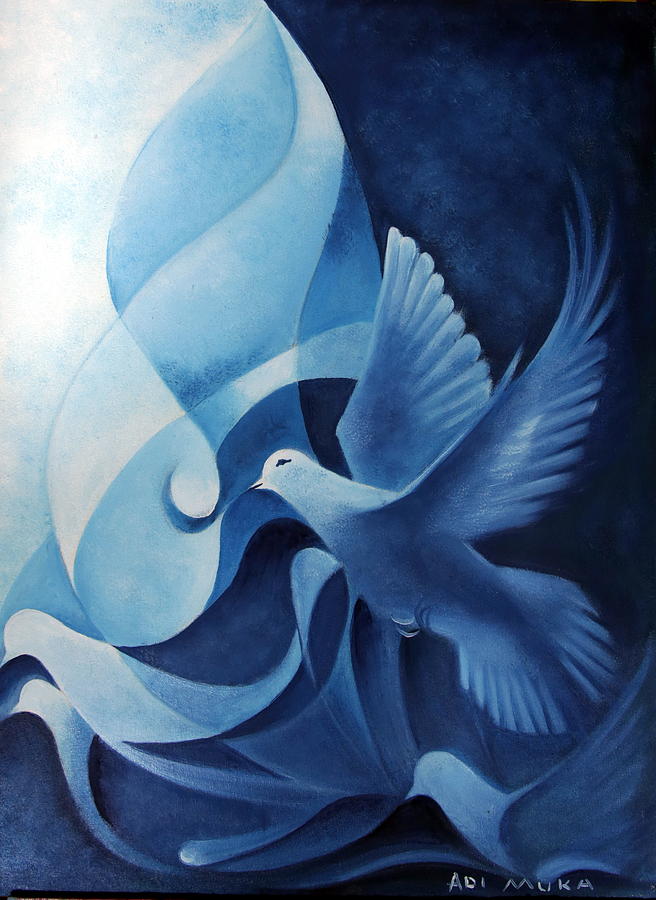This stunning artwork, created entirely in shades of blue, appears to be a pastel drawing or painting by an artist named Adi Muka, as indicated by the signature in the bottom right corner. The central focus of the piece is a magnificent dove in flight, illustrated in profile facing left. The white-faced dove, with its distinctive dark blue eye and delicate beak, spreads its wings upwards, revealing a mixture of white and blue feathers, and extends its fully fanned tail. The background transitions from dark blue on the right to a lighter, almost sky-like blue on the left, creating a mesmerizing gradient that swirls and curves throughout the canvas. Below the primary dove, there are visual echoes or silhouettes of birds in lighter blue hues, as if capturing successive moments in its flight. A spiral-shaped lighter blue element emerges from the tip of the dove’s beak, dissipating into the sky above and to the left, adding a dynamic and ethereal quality to the composition. The painting blends the abstract with the figurative, forming a harmonious and visually captivating piece.